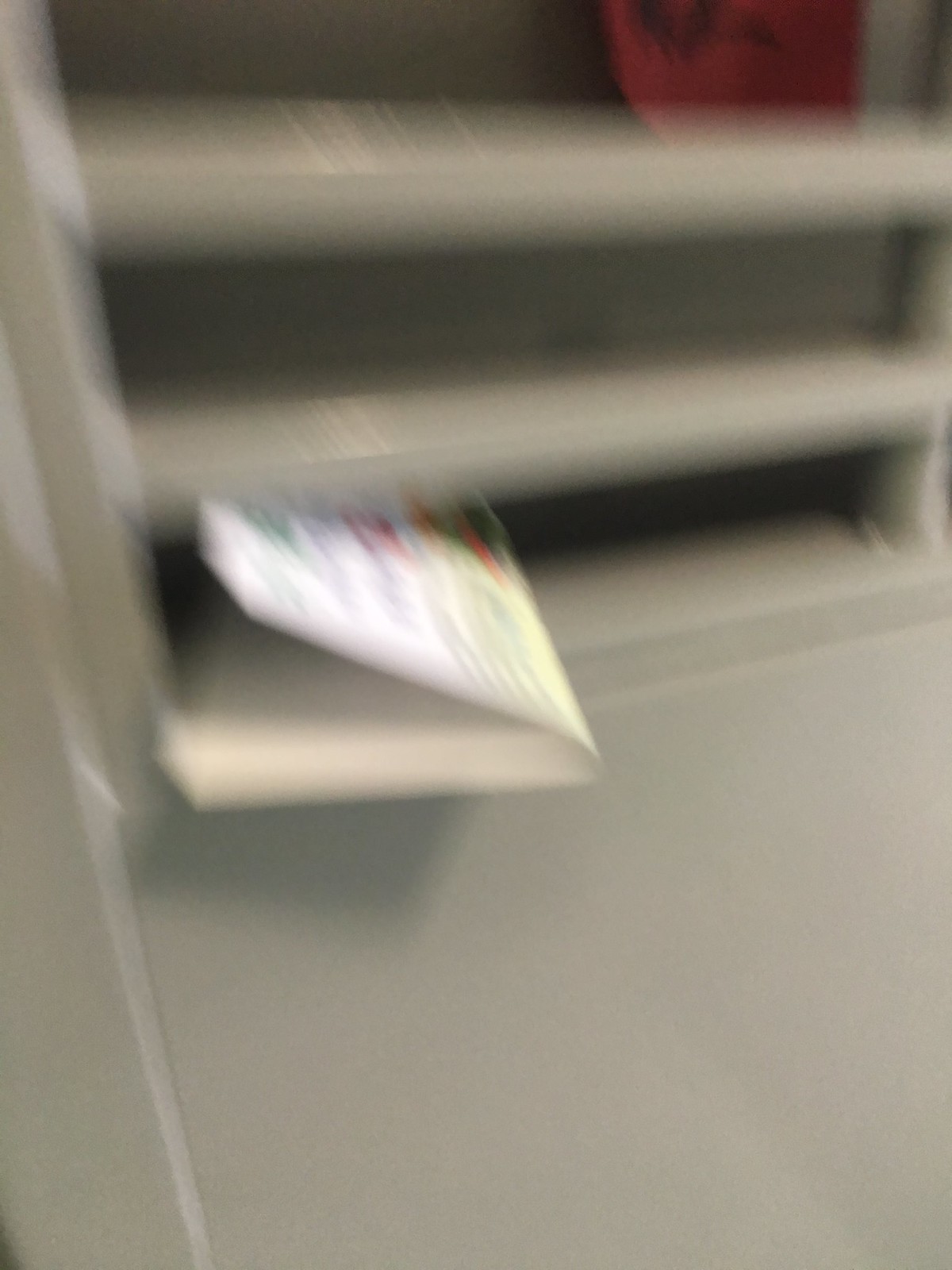This image, dominated by significant motion blur, features a wall or door structure with distinctive design elements. The lower portion is solid, while the upper section consists of slats or louvered windows. Wedged between the solid base and the first row of slats is a folded artifact; it's unclear whether this is an envelope or a piece of cardboard, but it displays some colorful markings on its surface. Through the slats, one can glimpse a background wall that appears dark gray. In the top right corner, there is a circular object, potentially a fire hose reel or fire hydrant.